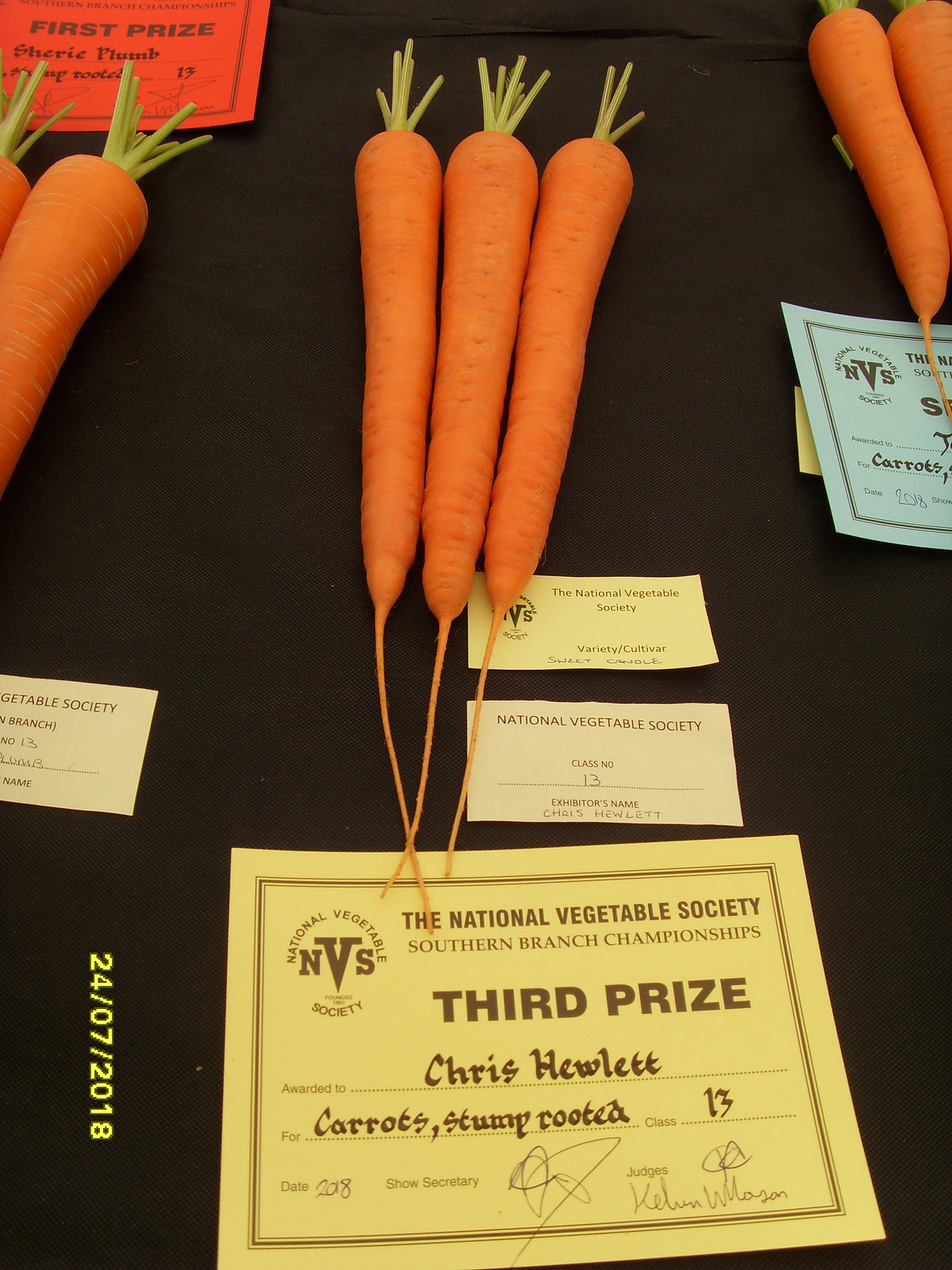This photograph captures an interior setting featuring a black cloth-covered table displaying prize-winning carrots. Central to the image are three long, orange carrots, celebrated for their quality with an array of certificates and ribbons. Underneath these carrots is a prominent yellow certificate indicating they earned third prize at the National Vegetable Society Southern Branch Championships, with exhibitor Chris Hewlett recognized for his stump-rooted carrots in class 13. The certificate spans the years 2008-2018, signed by both the show secretary and judges. Above the central carrots are additional National Vegetable Society cards detailing the variety and exhibitor's name, with the class number 13 noted. Flanking the main display are partial views of two other sets of carrots, one with a visible first prize ribbon. On the left side of the picture, other business cards can be seen, although some details are obscured. A vertical watermark dated 24-07-2018 is faintly visible on the bottom left of the photograph.